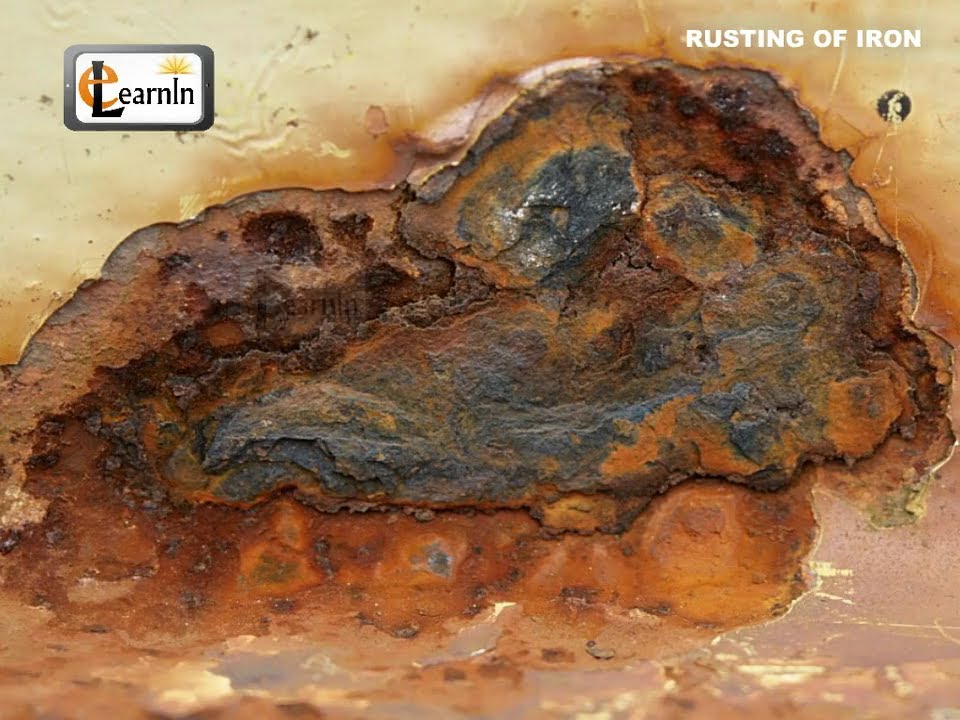The image depicts a close-up of a decaying and rusted piece of iron, characterized by a disturbed surface with jagged edges, holes, and patches of paint chipping away. The iron exhibits a variety of colors commonly associated with rust, including oranges, browns, grays, and whites, giving it a corroded appearance. In the upper left of the image, there is a logo featuring the words "E Learning" in a combination of black, white, and orange colors, with the design of the logo suggesting positivity and enlightenment, as indicated by sun rays emanating from the dot above the letter "I." In the upper right corner, the words "Rusting of Iron" are written in white font, highlighting the focal theme of the image. The overall backdrop is gray, complementing the varied tones of the rusted iron. The intricate details of the metal's decay and color spectrum contribute to the visual complexity and educational intention of the image.